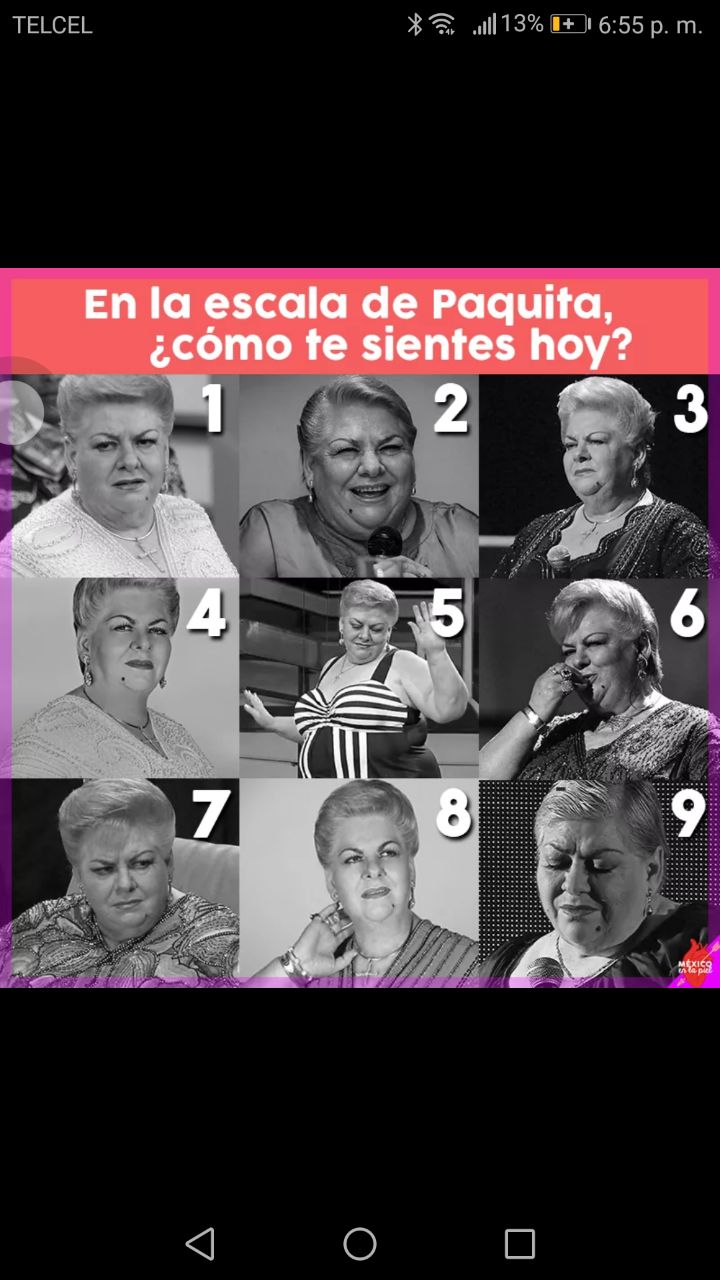The image is a screenshot taken from a phone at 6:55 p.m., with the Tell Cell network displaying full bars, Wi-Fi, Bluetooth, and a battery level at 13%. The caption at the top in red reads, "En la escala de Paquita, ¿cómo te sientes hoy?" which translates to, "On the Paquita scale, how do you feel today?" Below this caption, there are nine black and white photographs of a large, obese woman with short blonde hair, arranged in a 3x3 grid. Each photo captures her in different poses and moods. In one image, she wears a white dress and appears to be talking into a microphone; in another, she is in a black dress, looking left. Some photos show her wearing heavy jewelry, including earrings and rings. Notably, the center image depicts her wearing a bathing suit, and she seems quite cheerful. Other expressions range from staring off into the distance to looking very sad while speaking into a microphone. The background of the image has a purplish border with black at the top and bottom edges.